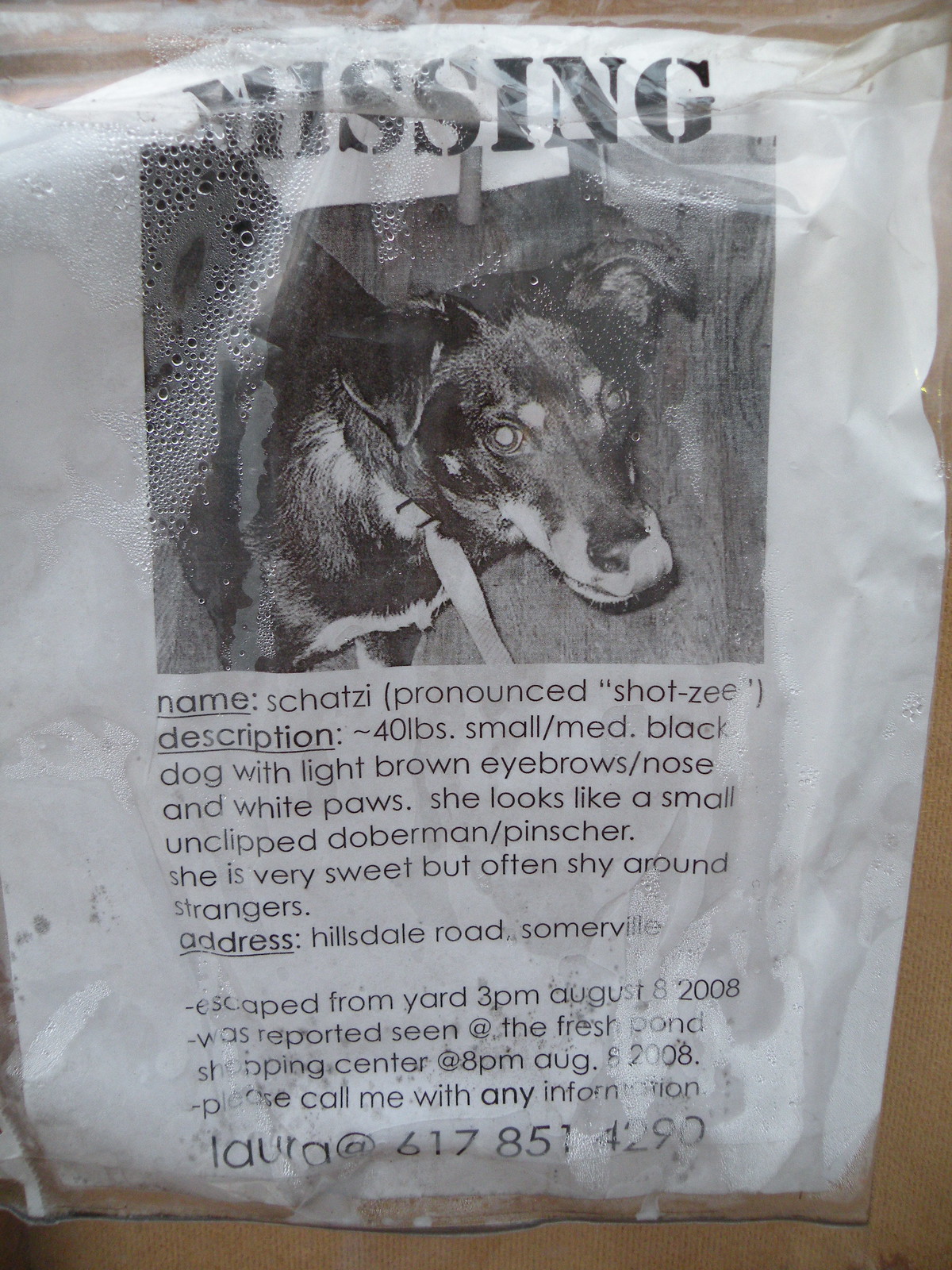This photograph depicts a weather-beaten missing dog sign, which appears crinkled and rain-damaged, enclosed in plastic with visible condensation. The sign is printed on a white piece of paper and features large, bold black font that reads "MISSING" at the top. Below that, there is a black-and-white image of the dog, a medium-sized black and white dog named Shotzi, who is described as weighing 40 pounds with light brown eyebrows, nose, and white paws. Shotzi resembles a small, unclipped Doberman Pinscher. The dog is noted to be very sweet but often shy around strangers. The sign also includes an address, Hillsdale Road, Somerville, and notes that Shotzi escaped from the yard at 3 p.m. on August 8, 2008, and was reported seen at the Fresh Pond Shopping Center at 8 p.m. the same day. For any information, it urges readers to call Laura at 617-851-4290. The sign appears to have been out in the elements for some time and looks like it had been posted and taken down, currently laying on a table.